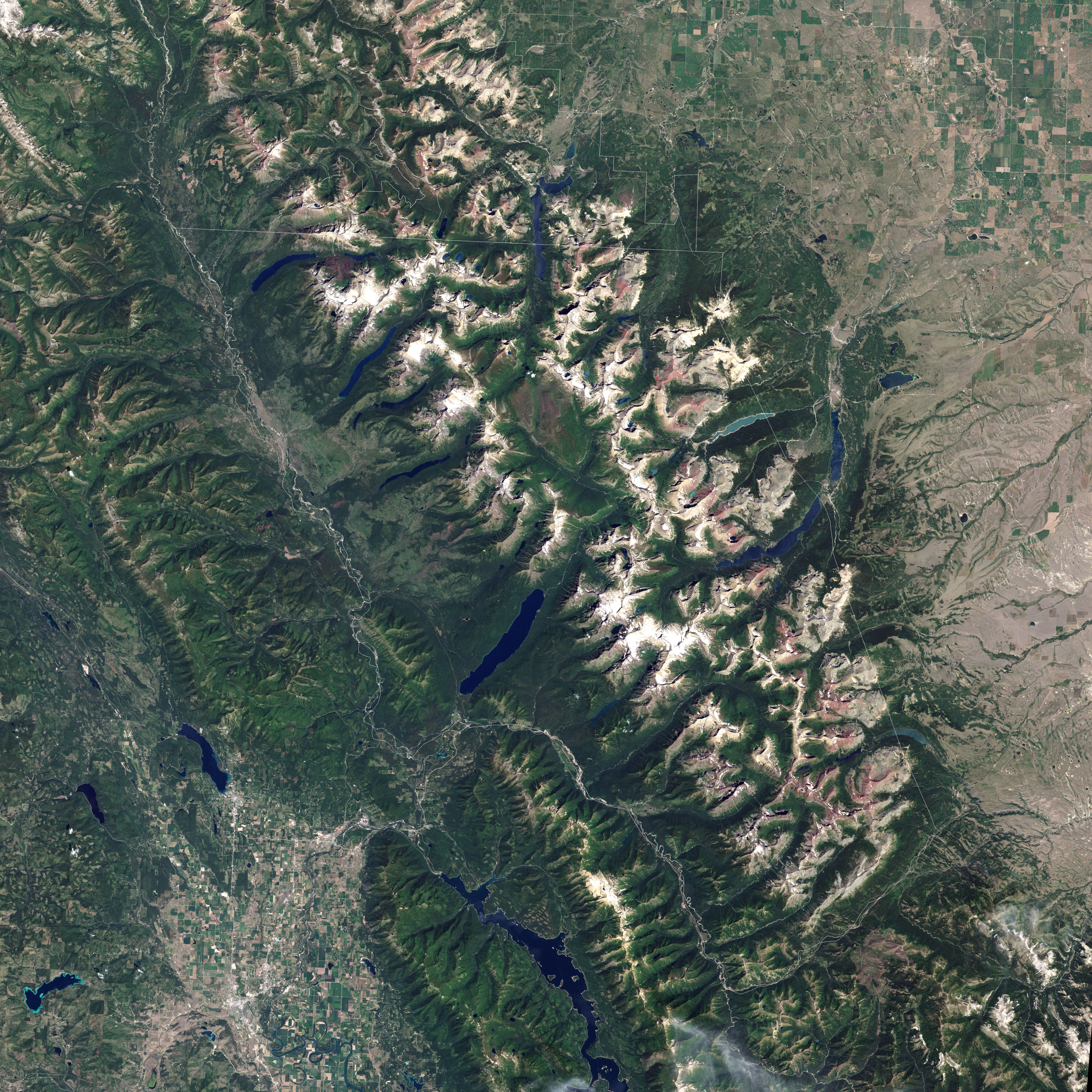This image, captured from a high altitude, provides a detailed aerial view of a diverse wilderness landscape dominated by a prominent mountain range running across its center. The peaks of this mountain range are capped in white, gradually transitioning to green and brown as the elevation decreases. On the right side of the image, the terrain is more arid, characterized by brown, cracked and dry areas interspersed with sparse greenery mainly at the hilltops, which appear less lush compared to the left side. 

In contrast, the left side of the image is replete with greenery, showcasing dense vegetation and multiple bodies of water, including a dark blue body in the bottom center and other small lakes towards the far left. Streams and rivers snake through the landscape, often flowing through the mountain range, contributing to the rich greenery in this region.

Further to the right of the mountain range, the landscape shifts to show patches of tundra and a more organized pattern of green squares, indicative of either houses or farmland plots, suggesting human habitation. A few small roads can be seen leading up to the mountains, possibly connecting these settlements. Additionally, in the southwest corner of the image, beyond the lush regions, there's a notable large light patch which might indicate a city, marking a stark contrast to the surrounding wilderness.